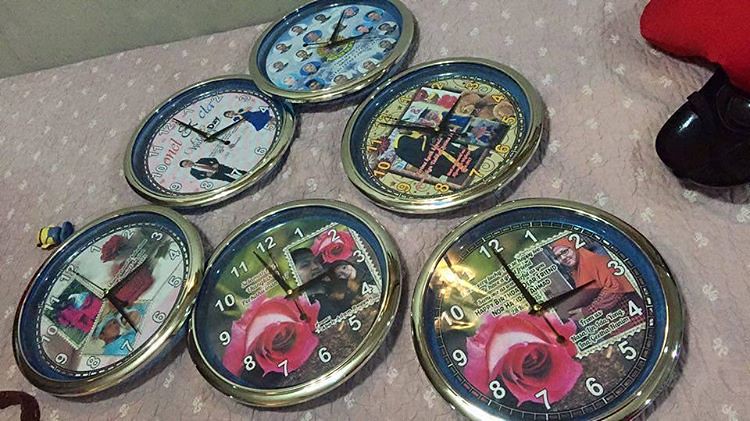This photograph, captured from a top-down perspective, prominently features six round analog clocks arranged in a pyramid formation—three at the bottom, two in the middle, and one at the top. Each clock showcases the traditional numbers 1 through 12, along with minute, second, and hour hands. Intriguingly, the faces of these clocks are adorned with various images: some feature portraits of people, including a woman in a red headscarf, while others display pictorial combinations of people and roses, accompanied by text, possibly names. The outer frame of each clock is golden, adding a touch of elegance to the display.

The clocks rest on a pink fabric surface dotted with white bows, possibly a bedsheet, lending a quaint backdrop to the scene. An angular black and red object can be faintly seen at the top right corner, its purpose indeterminate. The overall composition of this photograph draws attention to the intricate details of the clocks and the personalization of their faces, merging functionality with artistic expression.